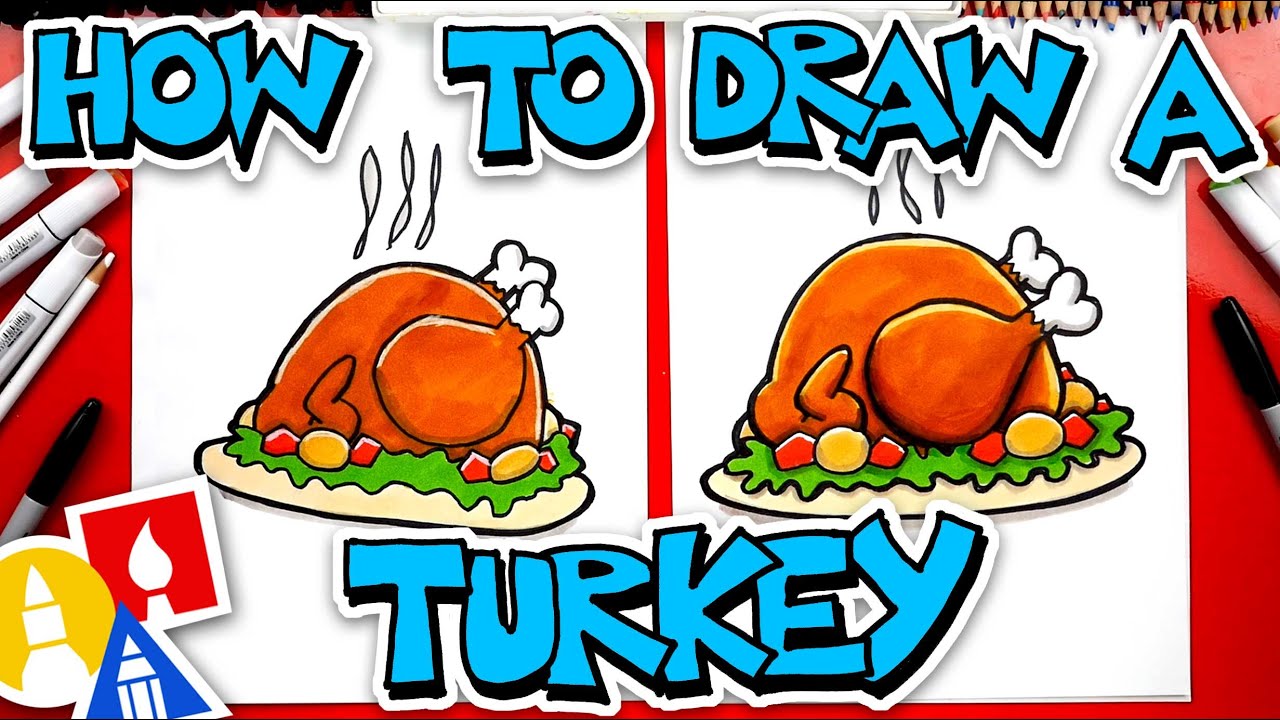This image is a detailed drawing tutorial titled "How to Draw a Turkey" in big blue letters outlined in black and white, placed prominently on a red background. The artwork features two cartoon-style, cooked turkeys resting on tan platters. The turkeys are brownish with white-ended drumsticks and are surrounded by decorative greenery, and small colorful vegetables that appear to be little fruits or potatoes, adding to the eye-catching visual appeal. Steam-like lines suggest the turkeys are hot. The background is divided down the middle by a red stripe, creating a neat, organized layout. The lower left corner showcases different drawing instruments—pens, a pencil, and a paintbrush—accompanied by blue, yellow, and red triangles indicating their usage. Emblems in red, blue, and gold add an extra touch of playful detail to the overall cute and comical design, emphasizing the instructional nature of the drawing.